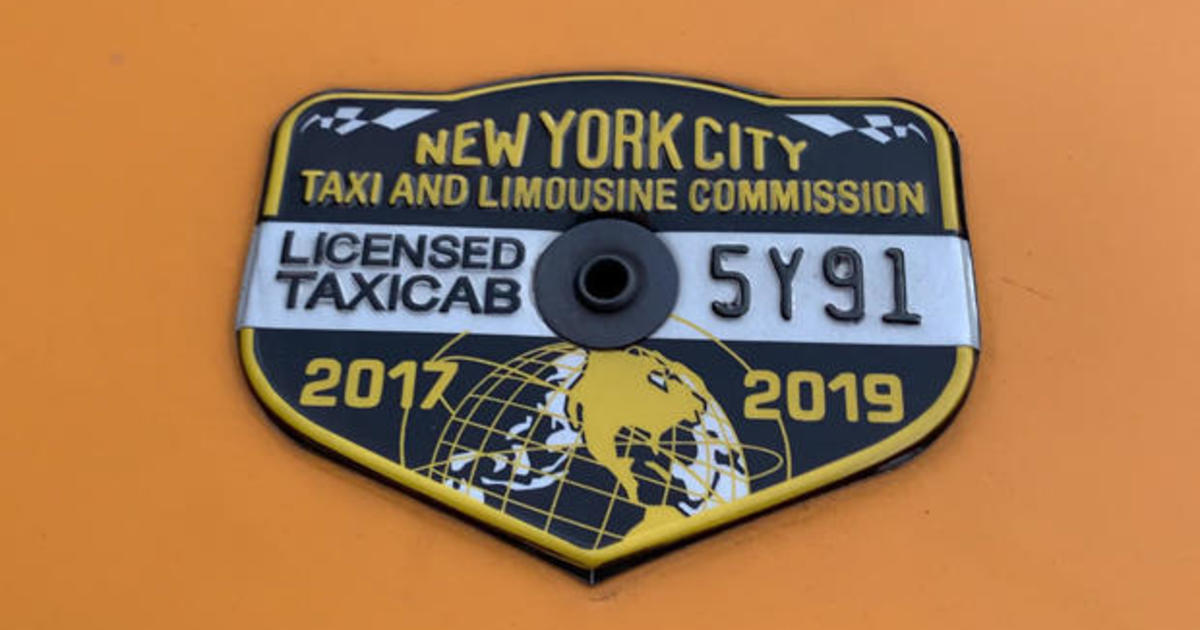The image features a detailed view of a taxicab license badge set against a vibrant orange background. The badge, primarily black with yellow accents, prominently displays "New York City" at the top in yellow lettering, beneath which it reads "Taxi and Limousine Commission." Below this, a silver banner is situated horizontally with bold black text: on the left, it states "License Taxicab," and on the right, it reads "5Y91," with a central black circular emblem, possibly a mounting fixture. In the lower section of the badge, the years "2017" and "2019" are inscribed in yellow on either side, flanking an image of the world outlined in yellow, showcasing North America. This badge appears to be an official decal likely attached to a yellow taxicab, representing its licensed status for the specified years.